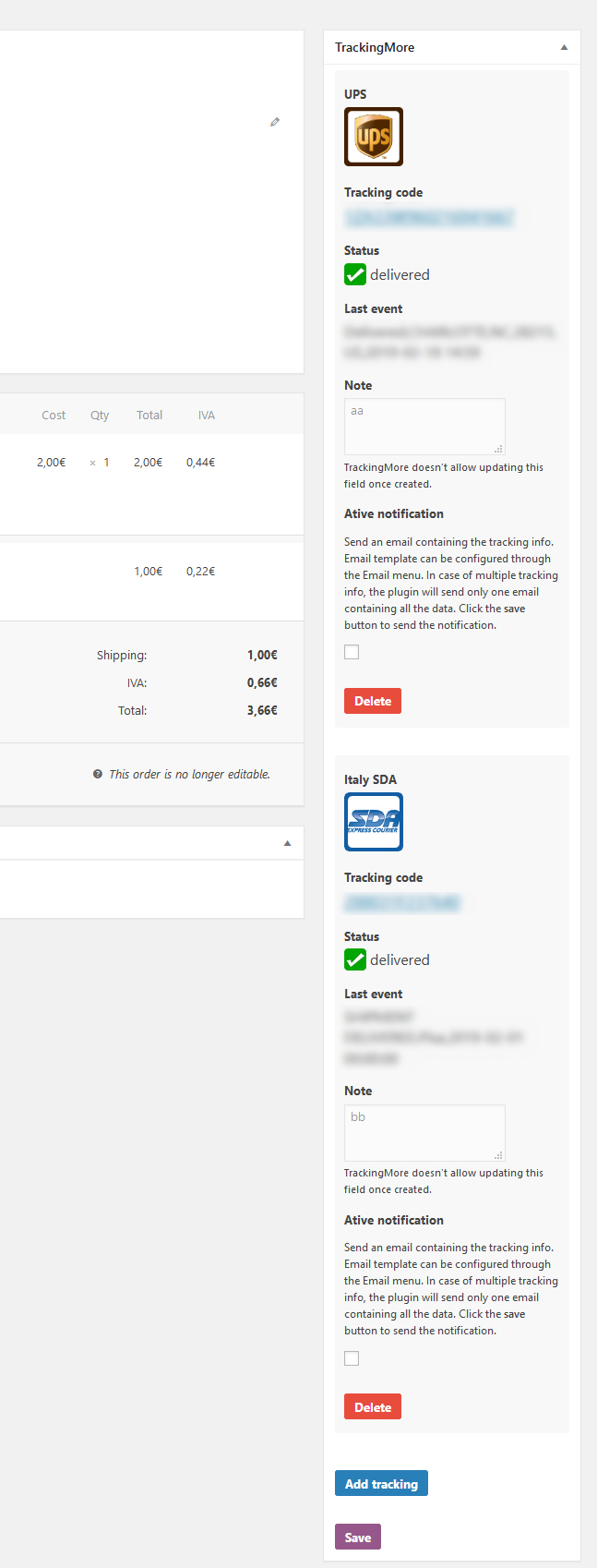The image appears to be a screenshot of a delivery tracking interface. At the top, the interface prominently displays the UPS logo, indicating the courier service used. The screen is divided into sections, with the right part providing detailed tracking information for multiple deliveries.

The first section mentions a package tracked via UPS, with its current status marked as "Delivered." Although the last event in the tracking history is blurred and unreadable, additional information like "Active Notification" is visible, albeit with small, indistinct text.

Below this, there’s another tracking entry for a delivery service labeled "SDA." This entry also shows a blurred-out tracking code and a status of "Delivered." Just like the previous entry, the "Last Event" and a note indicating "None" are present but unclear. An "Active Notification" is mentioned here as well, though the details are similarly hard to discern.

The interface continues with two buttons: a red button whose purpose is unclear from the description and a blue button labeled "Add Tracking." At the very bottom, there is a purple "Save" button.

On the left side of the screenshot, there is information regarding the shipping cost, which is denoted in pounds (£). The cost listed appears to be around £1.80 for shipping, with the total amount potentially in the range of £3. The specifics are somewhat difficult to read.

Overall, the screenshot details a tracking interface with multiple delivery statuses, notifications, and cost information, all set against a landscape of partially legible text and blurred-out details.